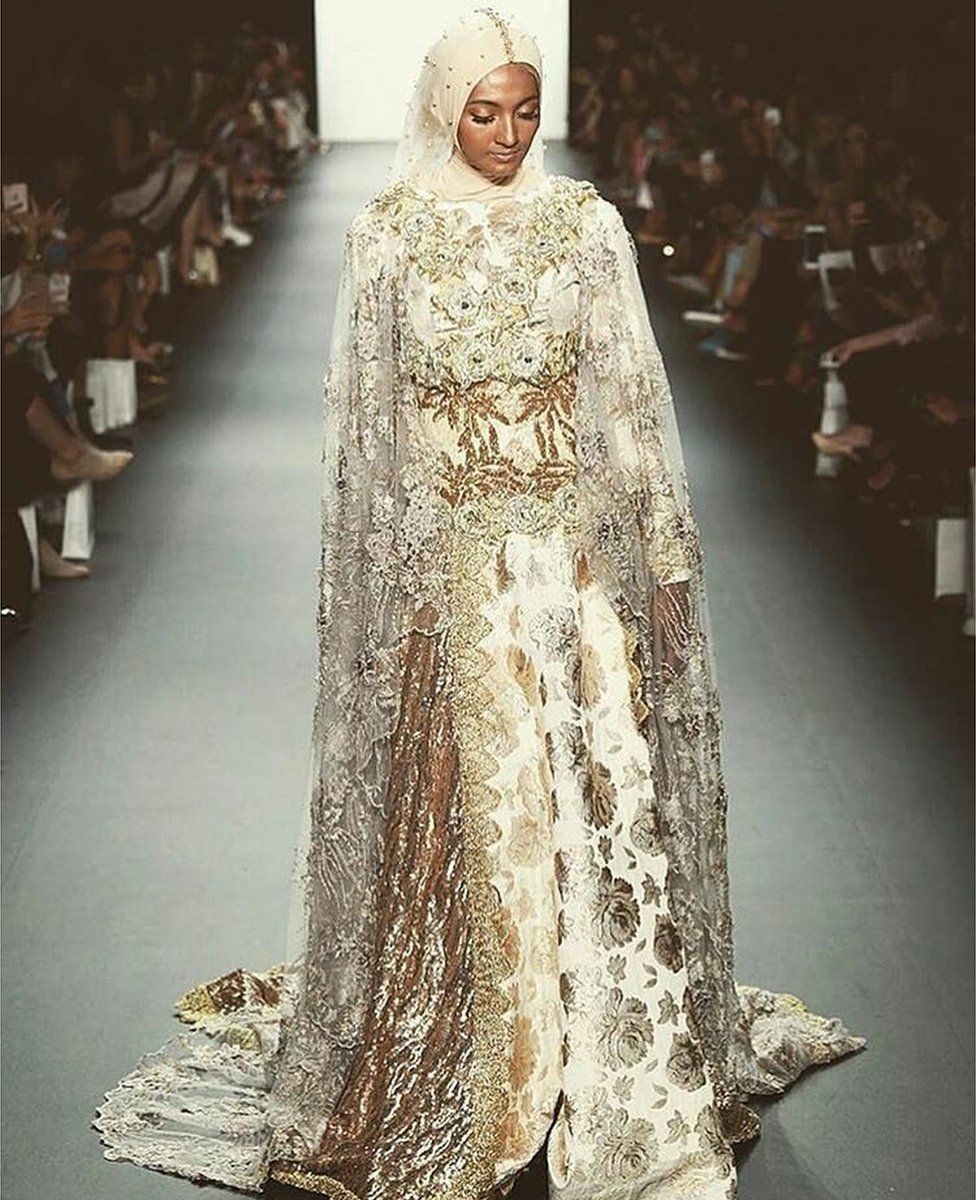The photograph captures a stunning moment on the runway where a model of dark brown skin is elegantly posed in an exquisite, flowing gown. The focal point of the image is the model, dressed in a lavish white and gold attire that appears to draw inspiration from traditional designs, possibly of Indian or Muslim origin. Her long-sleeved gown, rich with intricate gold and silver floral patterns and delicate lace, billows gracefully as she stands. The dress features ornate beadwork around the head, forming a headdress or scarf with gold beading, adding to the outfit's regal appearance. The gown drapes and converges into a pool of fabric at her feet, giving it a majestic aura.

The runway, illuminated by a bright white light, contrasts with the shadowed audience on either side, whose details are obscured but whose presence frames the model's path. Some audience members have gift bags at their feet and their forms, though not sharply defined, hint at their engagement with the show. The overall ambiance of the scene underscores the sophisticated and ethnic allure of the model’s attire, enhancing the photograph’s evocative depiction of high fashion.